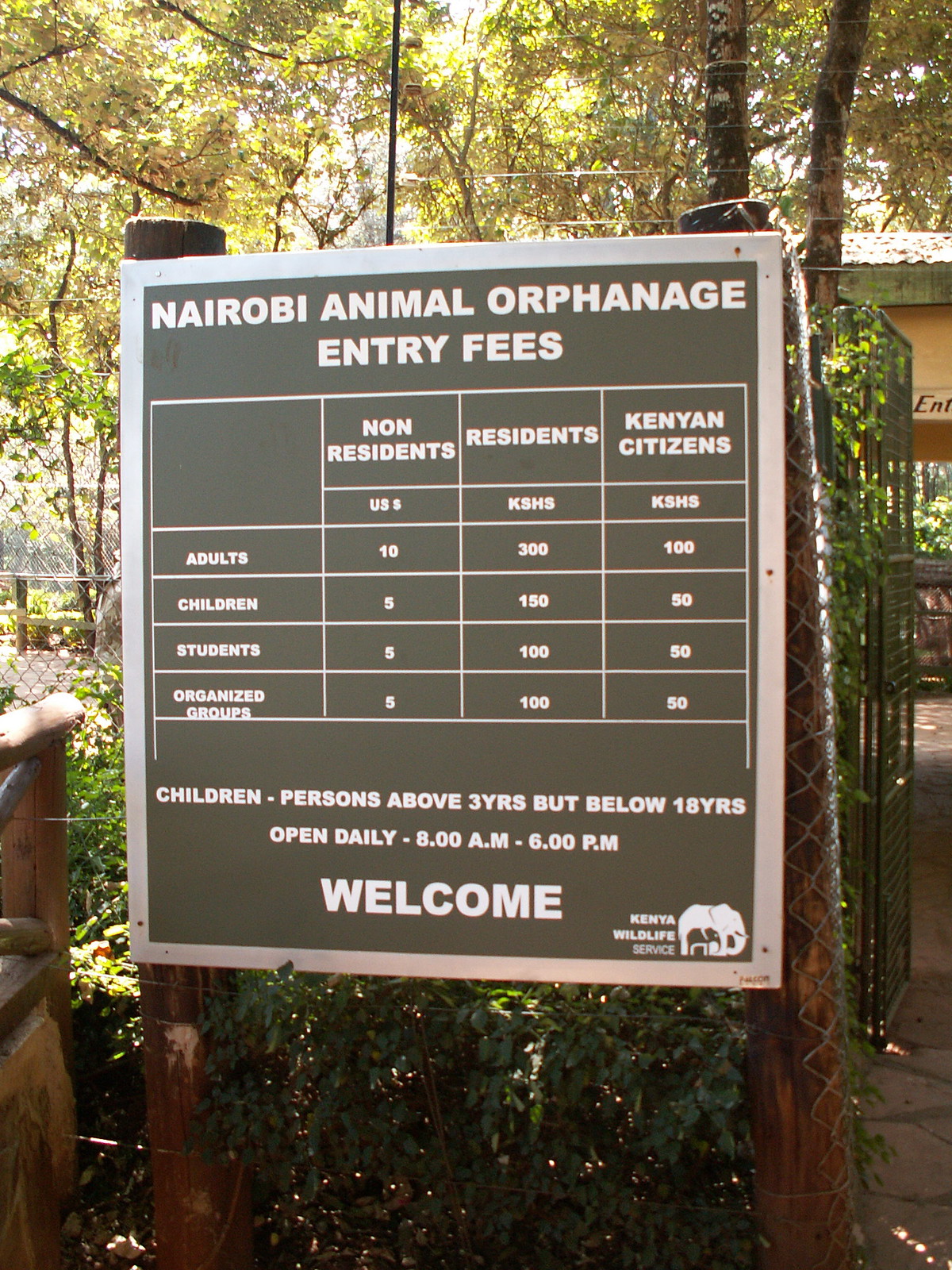The image captures a detailed scene at the Nairobi Animal Orphanage. Dominating the center of the frame is a prominent brown sign that lists the entry fees for various groups, including adults, children, students, and organized groups, with distinctions for non-residents, residents, and Kenyan citizens. The fee structure includes specific references to persons above 3 years but below 18 years. The sign also indicates the orphanage's operational hours, stating it is open daily from 8 a.m. to 6 p.m., and warmly welcomes visitors with a message from the Kenya Wildlife Service. In the bottom right corner of the sign, there is a small drawing of an elephant symbolizing the Kenyan wildlife. The background features a lush, vegetative landscape with various trees, bushes, and grass, indicative of an outdoor setting, likely in the middle of the day. A fence runs behind the sign, with glimpses of the orphanage on the right side and more trees on the left, enhancing the natural ambiance of the area. The colors in the image range from different shades of green and brown to splashes of white, black, and yellow, adding to the vibrant, earthy feel of the scene.